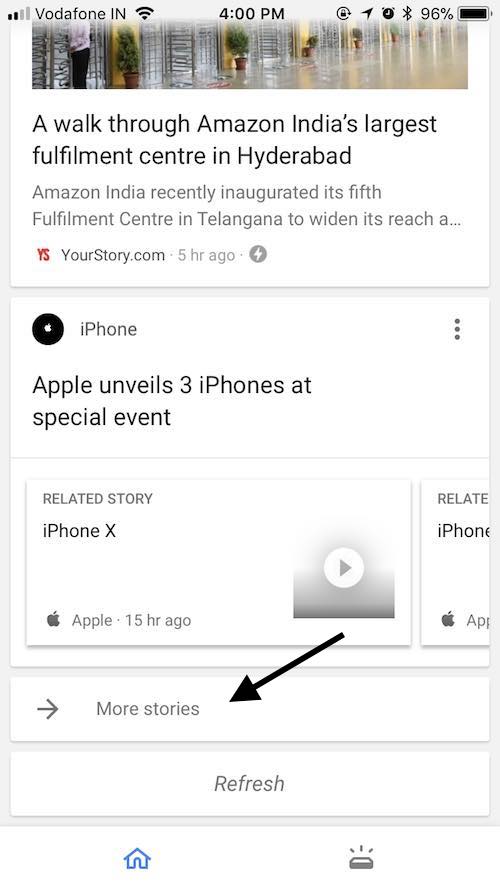This screenshot captures a mobile user's screen as they browse through what seems to be a news aggregation app, possibly on a browser. The top status bar displays various icons: a clock, the Vodafone IN network indicator, a signal strength icon, a Wi-Fi symbol, a battery icon showing 96% charge, and additional indicators including Bluetooth, an alarm, a lock, and a location icon.

Beneath the status bar, the browser's address bar shows the URL "yourstories.com." The main content features headlines such as "A walk through Amazon India's largest fulfillment center in Hyderabad" and "Apple unveils three iPhones at special event," with a related story mentioned as "iPhone X 15 hours ago."

At the bottom of the screen, navigation icons are visible, including a home button on the bottom left and a menu icon with three stacked lines. A darker arrow points to a "More stories" option, suggesting how users can access additional content. The phrase "Refresh here" is seen just below the main headlines, hinting that users can update the content feed.

The screenshot's top part appears cut off, making it challenging to confirm the exact app or webpage being viewed, as no company name or logo is visible. The overall simple interface allows users to browse and refresh various news stories efficiently.